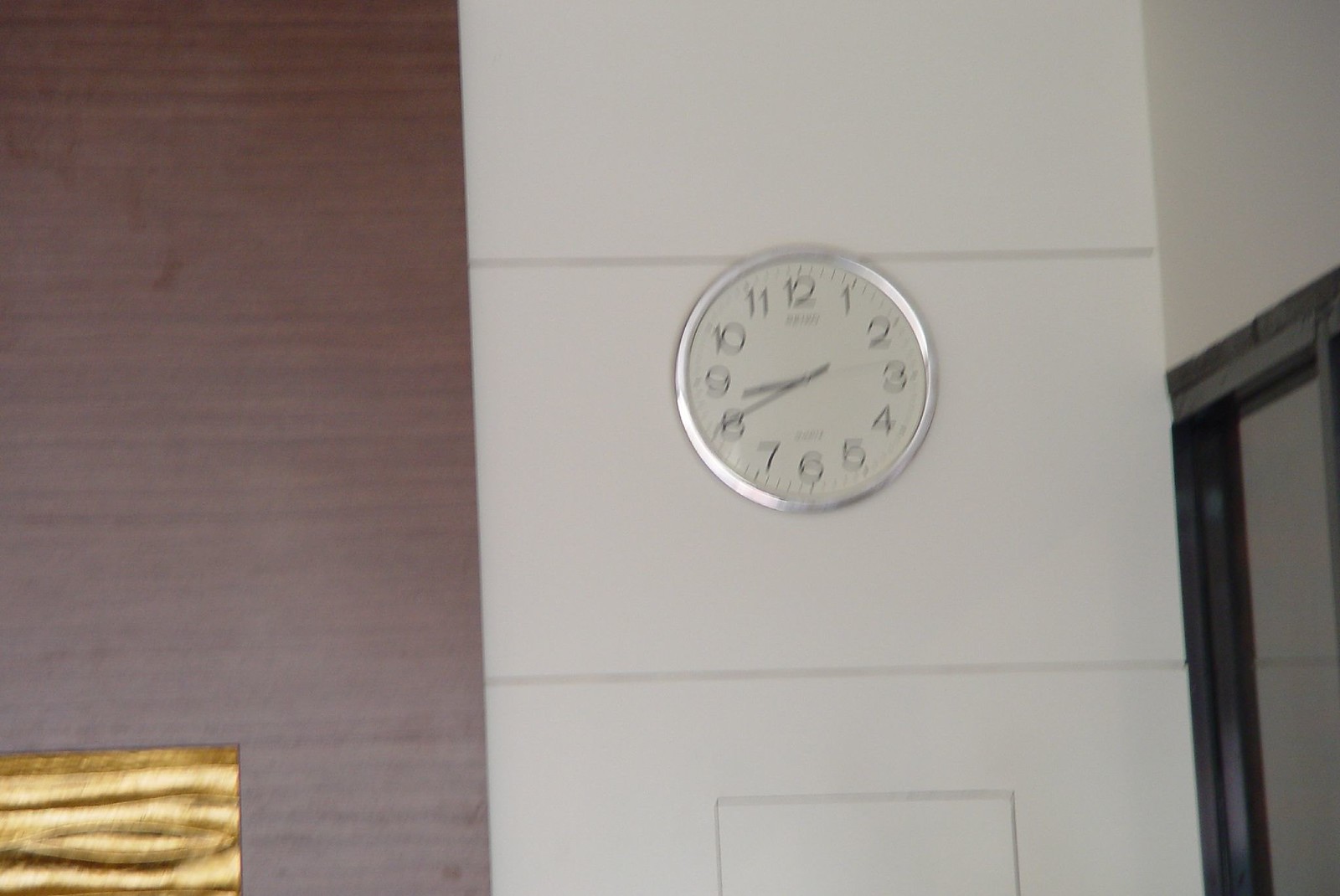The image depicts a room with two adjoining walls. The left-hand wall features a gradient of brown tones, transitioning from a dark brown at the top to a light gray-brown at the bottom. This wall is characterized by darker brown and black lines, adding texture to its appearance. In the lower left corner, there's an intriguing gold object, streaked with lighter and darker shades of gold, though its exact nature is indistinct.

The adjacent wall is primarily white and divided into three sections, each marked by horizontal gray lines. A clock adorns the middle section of this wall. The clock has a silver border with a white face, displaying black numeric digits and hands. The noted times vary slightly between 8:20 and 8:42. Further to the right, this white wall intersects with another section that houses a black-framed doorway. Inside the doorway, a gray door or possibly a translucent window can be seen. The overall scene might be set in a classroom due to its organized and structured layout.